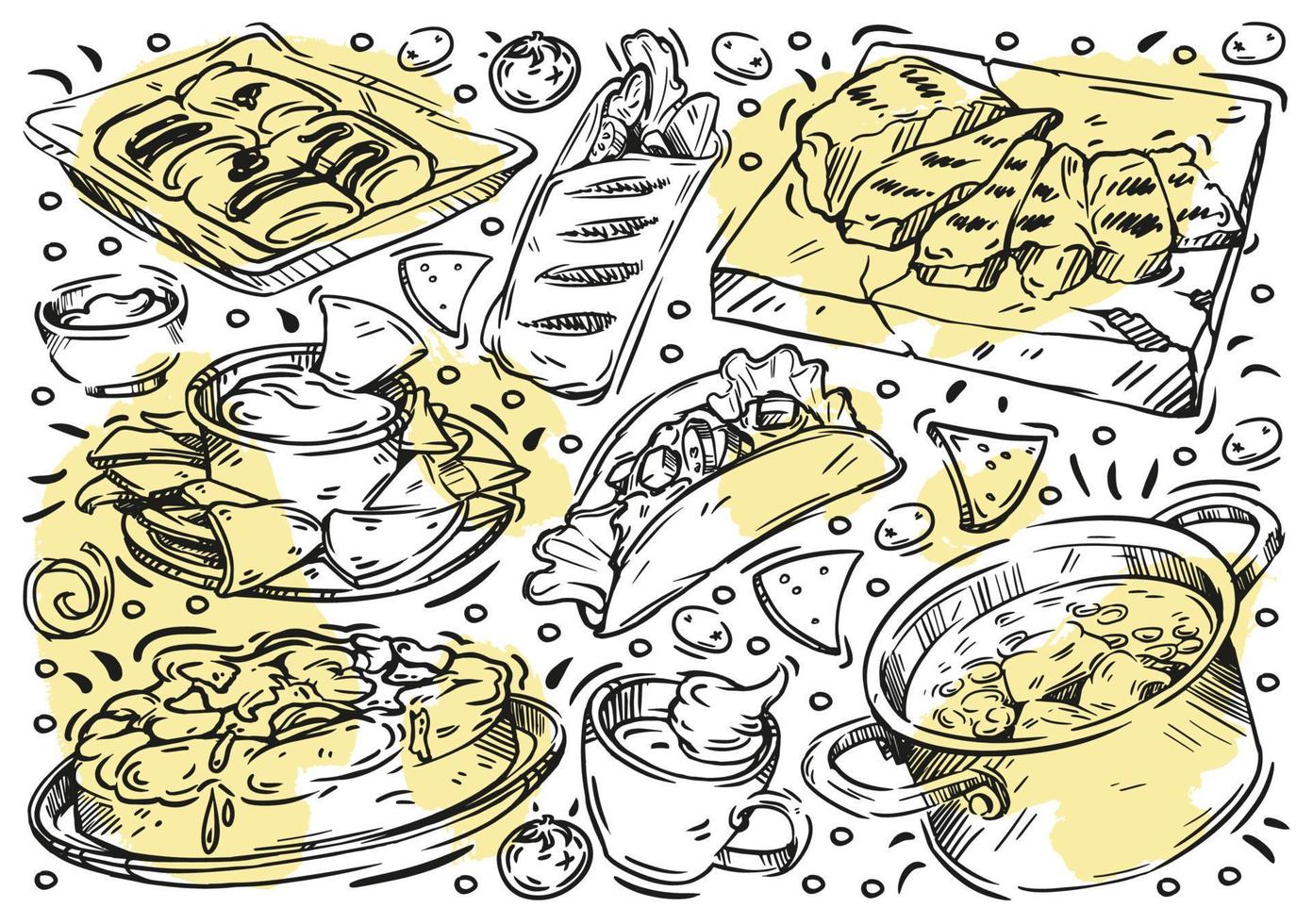This detailed black and white ink drawing appears to be set indoors and is filled with various foods, with some areas featuring intentional splotches of yellow. In the bottom right corner, a metal pot with two handles holds a yellow-colored dish. To the top right, there's a cutting board with six pieces of meat in various shapes, both triangular and rectangular. Adjacent to this is a bag of French bread. Beneath the meat, two triangular slices of pizza are shown. Moving left, there's a taco filled with vegetables just above a cup, likely containing hot chocolate topped with a dollop of cream. Close to this is a serving tray with what seems to be a mound of potatoes smothered in gravy. Above this, a dish of nacho chips accompanied by a bowl of dipping sauce is depicted. The top left corner houses a baking pan with four croissants, sitting directly above a bowl of what looks like butter. Scattered throughout the composition are small circles resembling tomatoes and sporadic black and white dots. The background integrates both white and tan hues, adding depth to the overall sketch.